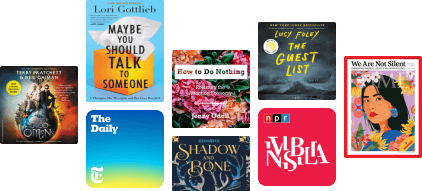This image is a composite screen capture featuring eight individual boxes, each showcasing a different podcast cover against a white background. Though the precise nature of these boxes—whether they are clickable links or merely advertisements—is unclear, they represent a selection of podcasts available on an unspecified platform.

1. The first box on the left depicts a podcast that appears to be titled "The Omen," featuring an image of two men sitting on a globe with a red fiery backdrop.
2. Next, a cover showcases a book by Lori Gottlieb entitled "Maybe You Should Talk to Someone," accented with an image of a tissue box with white tissues, reminiscent of a book cover.
3. Below that, a recognizable podcast called "The Daily" from The New York Times is represented with a gradient blue-to-green background, featuring the iconic stylized "T."
4. Another box presents a cover with a vibrant floral pattern and the title "How to Do Nothing," although the author's name is partially legible as Jenny Odette.
5. The following box displays a dark, visually striking cover of "Shadow and Bone," with a black background interspersed with bone imagery.
6. The fourth column highlights "The Guest List" by Lucy Foley within a box that features a cloudy night sky with a full moon, accompanied by a handwritten font.
7. A red square in the fifth box features the NPR logo in the upper left corner, but the podcast title is difficult to decipher.
8. Finally, the last box portrays a colorful, stylized depiction of a woman with long dark hair surrounded by flowers on a purple background, labeled "We Are Not Silent."

The image collectively showcases these diverse podcast offerings, each standing out through distinct visual art and typography.